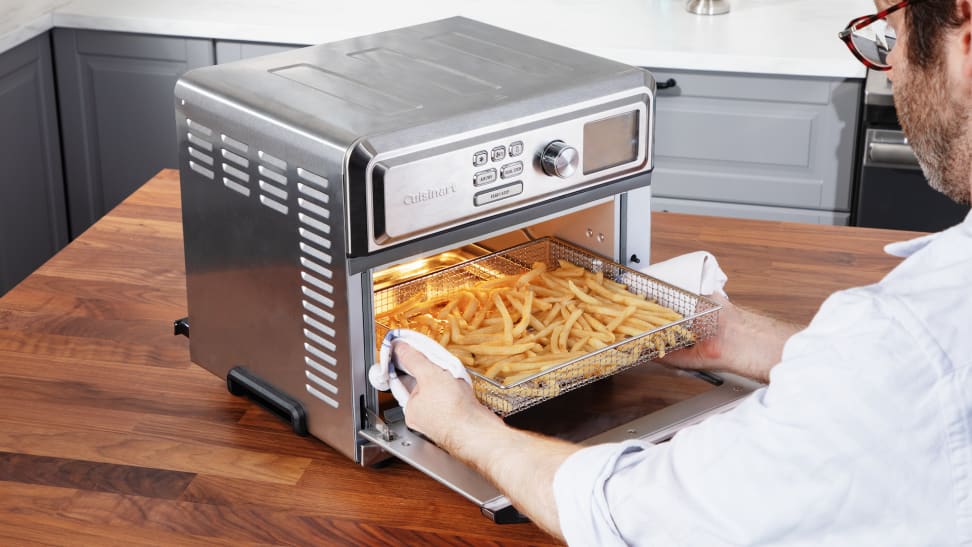The image features a close-up of a stainless steel Cuisinart toaster oven situated on a large butcher block-style wooden countertop island. The toaster oven, which resembles a small air fryer, has a set of controls on its front: three square buttons at the top, two rectangular buttons below them, and a wide rectangular button below those, alongside a knob and a digital screen on the right. The device, prominently silver-colored, stands out at the center of the landscape-oriented photo.

To the right side of the image, a man with glasses and a slight beard is visible, partially showing the left side of his face. He is wearing a white shirt and uses a towel to handle a mesh wire tray filled with potato fries, which he appears to be either sliding into or pulling out of the oven. The scene's background shows gray and white cabinets, adding context to the kitchen setting.